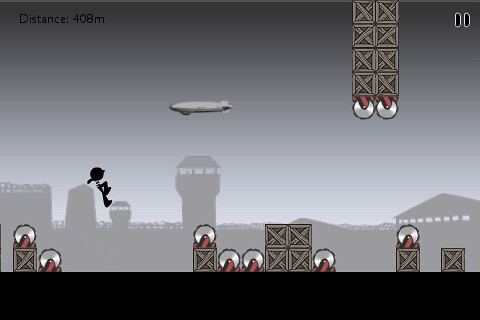In this dynamic video game scene set in an airport, the atmosphere is dominated by a foreboding gray sky that darkens towards the top of the screen, suggesting an impending storm or dusk. A sleek, silver airplane slices through the air, flying directly over a towering structure that appears to be an air traffic control tower, a critical hub for managing aircraft movements. Surrounding the tower are various airport buildings, creating a bustling backdrop indicative of a lively, operational airfield.

In the foreground, a series of spotlights mounted on wooden boxes are prominently featured. These brown wooden boxes serve as sturdy platforms for the lights, which are firmly secured with red fixtures. The spotlights themselves emit a bright, clear white light, possibly illuminating the runway or guiding the airplane's approach. This meticulously detailed setup adds to the immersive, high-stakes environment typical of a video game airport scene.